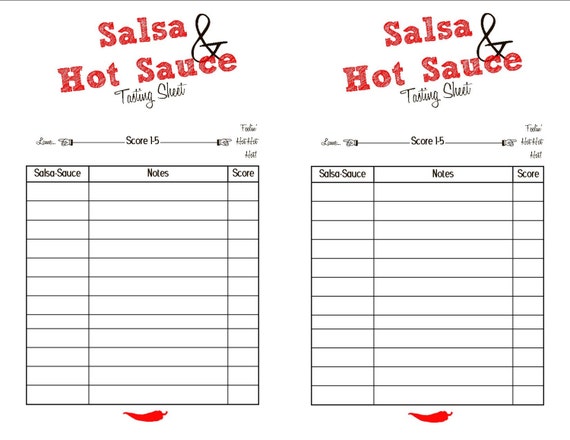The image is a horizontally aligned rectangular sheet, white in color, used as a tasting sheet for salsa and hot sauce. It features two identical sections side-by-side. At the top of each section, "Salsa & Hot Sauce Tasting Sheet" is prominently displayed in red letters, while "tasting sheet" is written in black cursive underneath. A thin gray horizontal line runs across the very top of the sheet. Below the title, each section contains a table divided into three columns labeled "Salsa - Sauce," "Notes," and "Score," from left to right, with "Notes" being the widest column. The table is comprised of approximately 10 empty rows for recording data. At the bottom center of the sheet, underneath the tables, there is a small drawing of a red chili pepper.